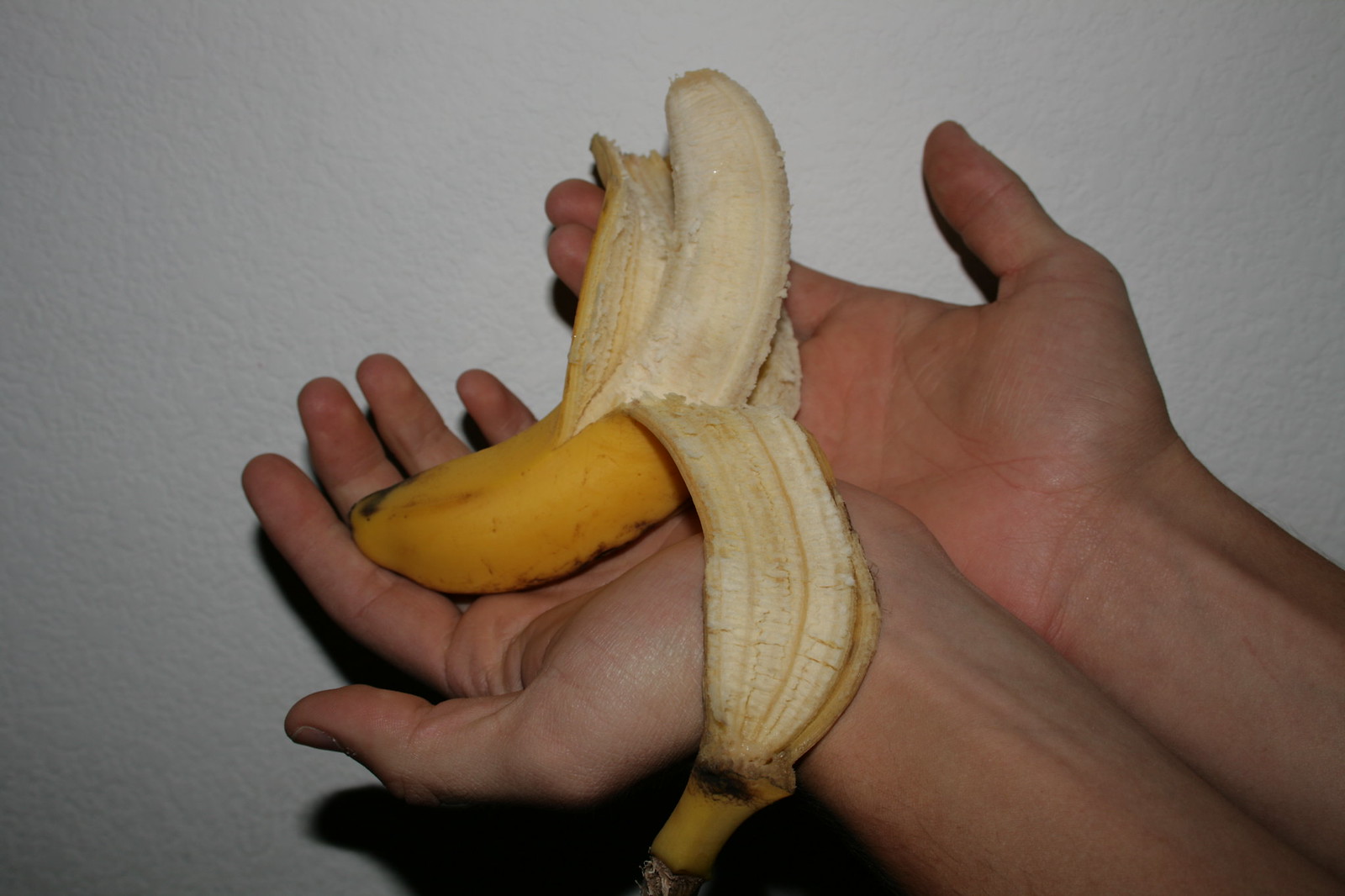The image showcases a simple yet striking scene against a rough, white wall that bears several cracks, providing a textured backdrop. Dominating the center of the composition is a peeled banana, its vibrant yellow skin accented with a few black marks on the top, bottom, and sides. The inside of the banana is a pale whitish color, blending seamlessly with its modestly hued peel. Supporting the banana are a pair of hands, visible from the fingers to the wrists, positioned diagonally in the lower right section of the frame. The skin tone of the person holding the banana is light, and the fruit rests delicately on the ends of their fingers and middle palms. Notably, the peel drapes over the left wrist and makes contact with the pointer finger on the right hand, emphasizing the gentle grip and the natural, relaxed posture of the hands.